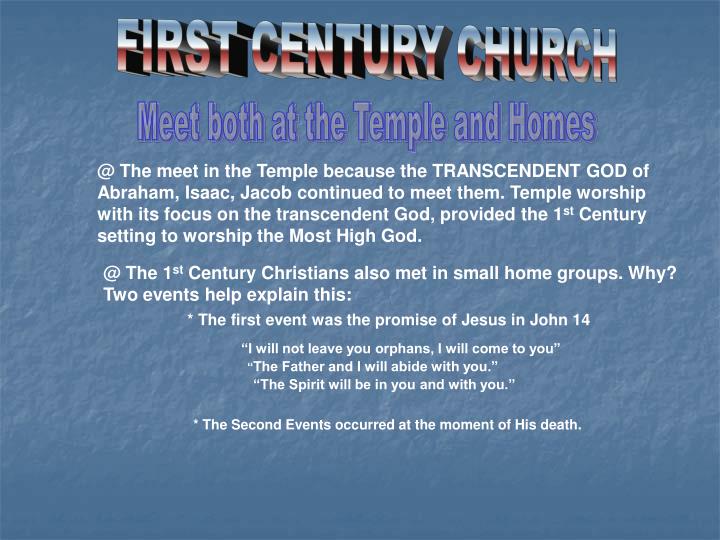The image is a digital advertisement resembling an HTML webpage, centered around the theme of the "First Century Church." It features a medium blue background that has a subtle, lightly textured effect giving it a three-dimensional quality, most prominent in the center and fading towards the edges. At the very top, the main title, "First Century Church," is rendered in a bold, capitalized block font with a metallic gradient transitioning from blue at the top to red at the bottom. Beneath this title, a subtitle in purple states, "Meet both at the temple and homes."

Further down, the text elaborates on this theme in white font. It explains that first-century Christians met in the temple to worship the transcendent God of Abraham, Isaac, and Jacob, emphasizing that temple worship provided the setting to worship the Most High God. Additionally, it details that Christians also gathered in small home groups. To explain this dual meeting practice, two key events are highlighted. The first event is a promise from Jesus in John 14, quoted as, "I will not leave you orphans; I will come to you. The Father and I will abide with you; the Spirit will be in you and with you." The second event occurred at the moment of Jesus's death, underscoring the profound changes in early Christian worship practices.